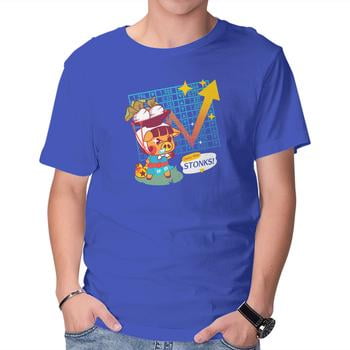This image features a young man wearing a blue t-shirt adorned with a detailed graphic on the front. The subject's face is not visible, only a portion of his chin is shown, and the image extends to his hands, which are tucked into his pockets. On his left wrist, he wears a bulky watch with a black leather strap, while a silver and black bracelet adorns his right wrist. 

The prominent graphic on the t-shirt captures a blend of whimsical elements: it prominently features a character from Animal Crossing, often associated with the turnip trade, wearing a turquoise dress and a kerchief. The character, which resembles a pig dressed with a bowl of turnips on its head, carries a bag of bells, a staple item from the game.

Behind the character is a grid background complete with charts, numbers, and stars, accentuated by a multicolored line graph that fluctuates and ultimately points upwards, symbolizing rising trends. Beside this graphical representation is a speech bubble that emphatically says "STONKS!" in large, bold letters. This humorous and detailed design brings together elements of video game culture, financial parody, and playful aesthetics in one unified image, much like you'd find in a catalog.